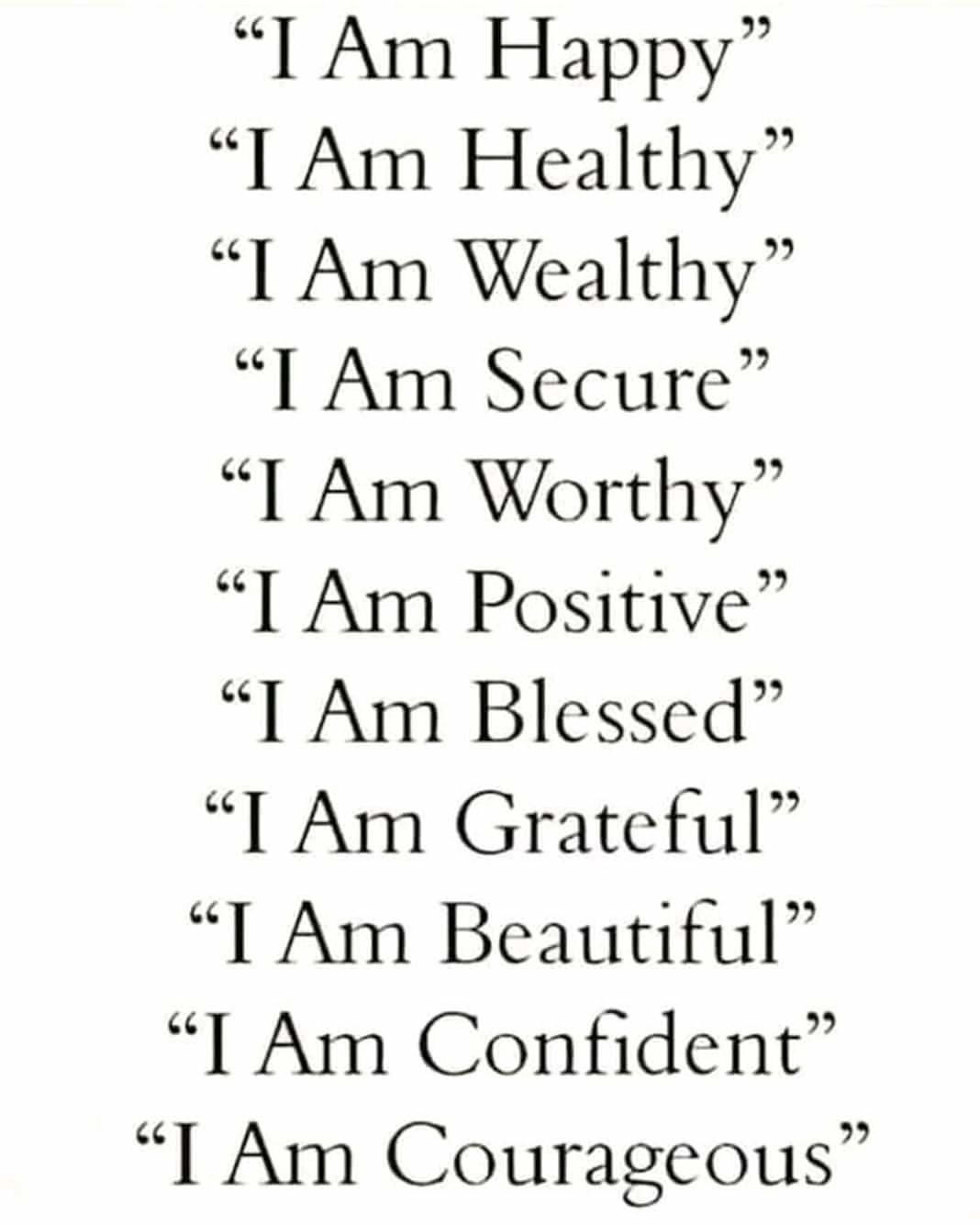The image is dominated by a large, centered wall of text on a white background, featuring a series of self-affirmations. Each line starts with "I am" and includes phrases like "happy," "healthy," "wealthy," "secure," "worthy," "positive," "blessed," "grateful," "beautiful," "confident," and "courageous." The text is in bold, black font with consistent capitalization of the first letter in each word. The affirmations extend from the top to the bottom of the image, taking up almost the entire vertical space, with just a bit of empty space on the left and right sides. There is no border, and the motivational style suggests it is intended for sharing on social media platforms. The colors in the image are primarily white and black, with a hint of light brown.